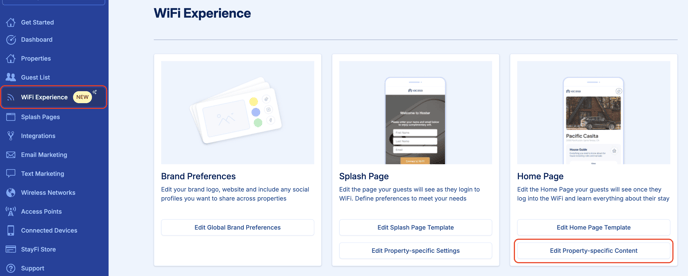The image captures a comprehensive Wi-Fi settings management page within an administrative dashboard. 

At the top left corner, several navigation options are visible, including "Get Started," "Dashboard," "Properties," "Guest List," along with what appears to be an active section related to "Wi-Fi Experience." A prominently placed "New Tool" button suggests functionalities for enhancing user management.

The main content area is dedicated to various Wi-Fi management tools. These include:
- "Splash Pages" where administrators can configure the introductory page guests see upon logging into the Wi-Fi.
- "Integrations" for connecting with various services.
- "Email Marketing" and "Text Marketing" for communication purposes.
- "Wireless Networks" to manage network settings.
- "Access Points" and "Connected Devices" for hardware and device management.
- "Stay Fiest" or "Support" options for assistance and troubleshooting.

The central portion of the page emphasizes "Wi-Fi Experience," featuring three key sections each illustrated with images. 

1. **Brand Preferences:**
   - Descriptive text prompts administrators to edit their brand logo, website, and include any social profiles to share across properties.
   - Options include "Edit Your Brand Preferences" and "Edit Global Brand Preferences."

2. **Splash Page:**
   - Administrators can customize the initial page that guests see when logging into the Wi-Fi.
   - Text advises defining preferences to meet specific needs, with options to "Edit Splash Page Template" and "Edit Property Specific Settings."

3. **Home Page:**
   - This section focuses on the page guests are directed to once they log in, providing them with information about their stay.
   - Available actions include "Edit Home Page Template" and "Edit Property Specific Content."

The detailed interface suggests a robust platform designed for intricate management of Wi-Fi network experiences, catering to customization at both global and property-specific levels.